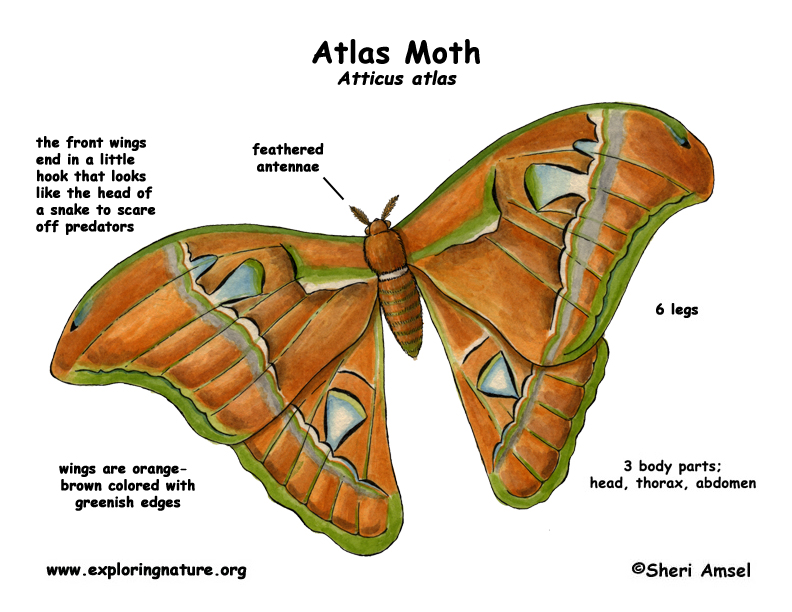The image is an illustrated diagram of an atlas moth, scientifically known as Atticus atlas, featuring detailed annotations about its anatomy and characteristics. The title "Atlas Moth" is prominently displayed at the top in black text, followed by its Latin name. The illustration showcases the moth in a rich, deep orange-brown hue with intricate greenish edges outlining its large, triangular wings, which also feature white and blue splashes. 

Annotated labels describe various parts of the moth: its feathered antennae are highlighted, and the front wings are noted to end in a hook resembling a snake's head, a defense mechanism to deter predators. The diagram also details the moth's six legs and its three main body parts: the head, thorax, and abdomen. Additionally, a watermark at the bottom right credits Sherry Amsel and the website www.exploringnature.org. Overall, the image combines both visual and textual elements to provide an informative look at the atlas moth's distinct features.